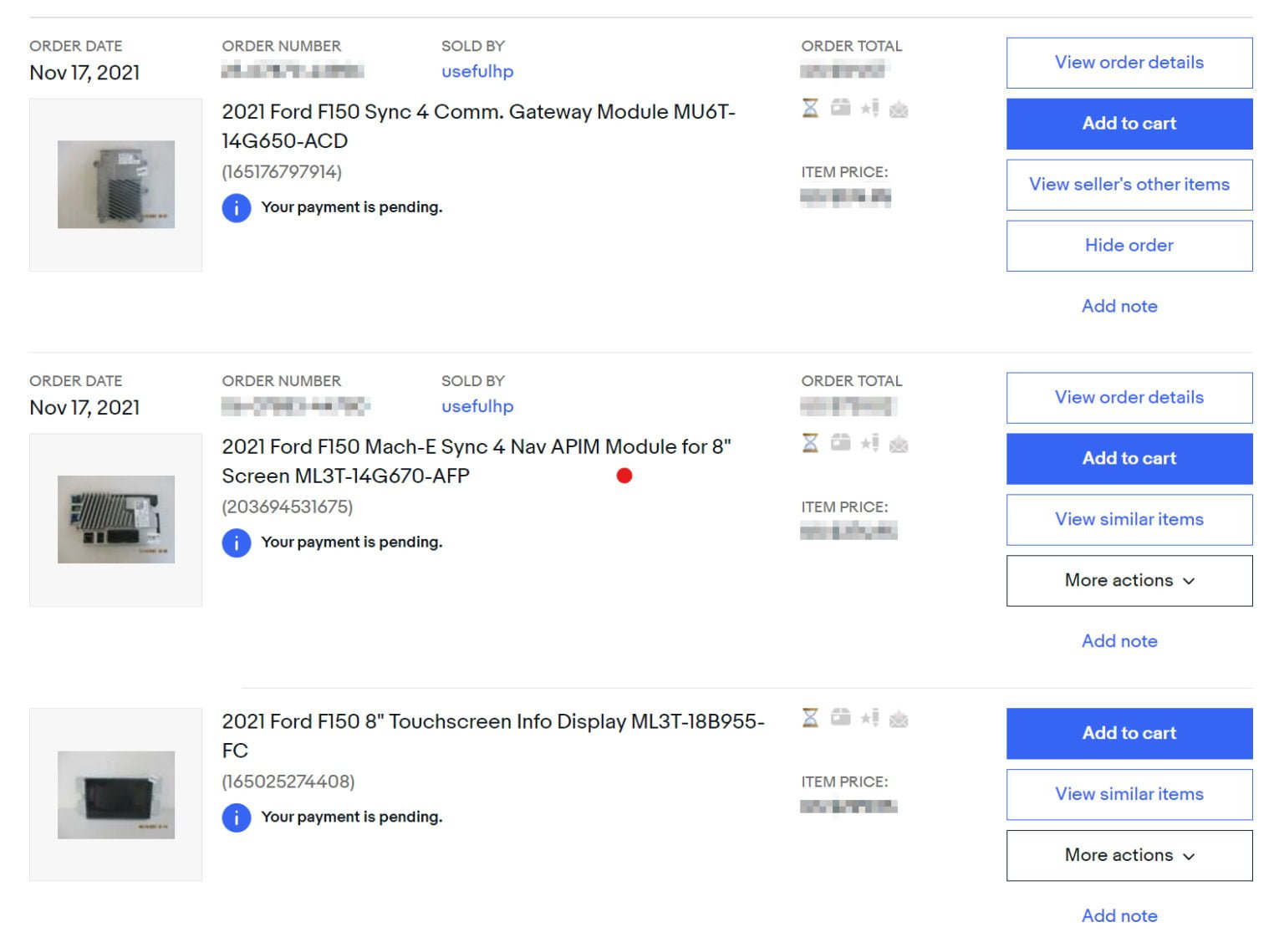A detailed caption for the image could read:

"Screenshot of a webpage displaying order details. In the top left corner, 'Order Date' is prominently displayed, indicating November 17th, 2021. This date appears consistently in adjacent images as well. At the very top, the 'Order Number' is shown but has been blurred for privacy, along with the total order amount. 

The primary focus is on the first two listed items, both sold by 'Useful HP.' Specifically, the items are described as '2021 Ford F150 Sync 4, Gateway Module MU6T.' An important note on the page indicates that the payment status for these items is currently 'Pending.' The interface provides options to 'View Order Details,' 'Add to Cart,' 'View Seller’s Other Items,' and 'Hide Order,' offering user-friendly navigation for further actions."